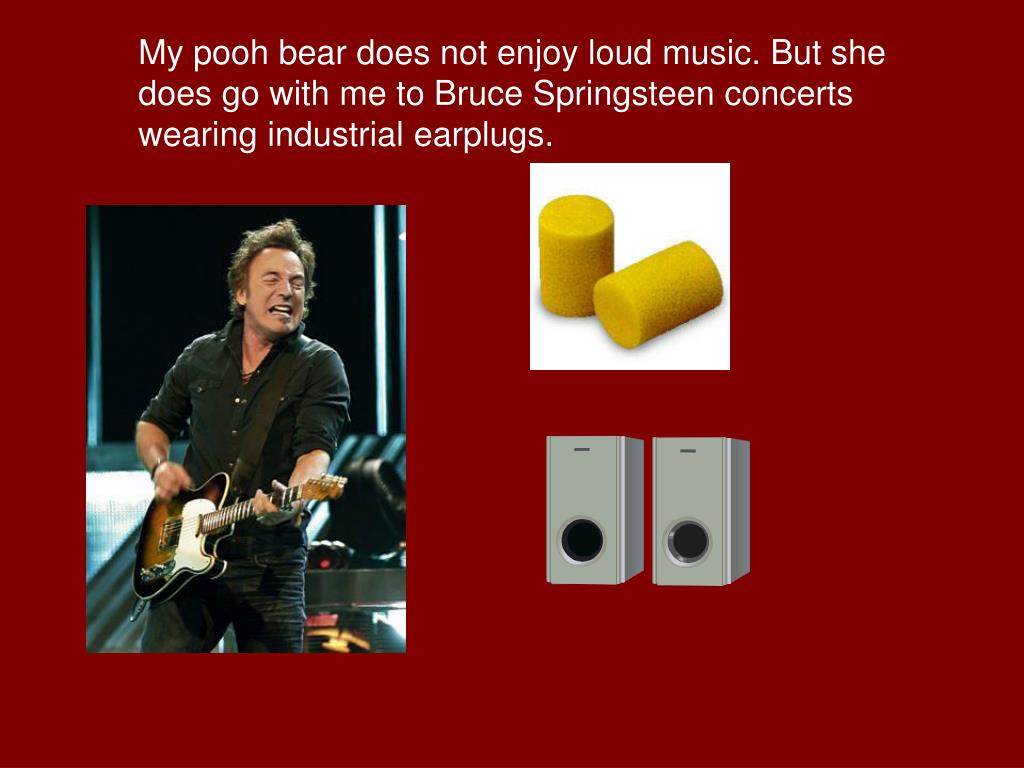The image features a dark maroon background with a white caption at the top in Arial font, reading: "My pooh bear does not enjoy loud music, but she does go with me to Bruce Springsteen concerts wearing industrial earplugs." On the left side of the image, there's a photograph of Bruce Springsteen, a middle-aged white man with unkempt brown hair. He's wearing a black polo shirt and black pants, carrying a brown and white guitar while gritting his teeth, suggesting he is intensely involved in his performance. To the right of Springsteen's photograph, there is a white square containing two yellow, foam, cylinder-shaped earplugs—one standing upright and the other lying on its side. Below this square are two silver speakers with large black circles towards the bottom, indicating the sound output area. Behind Springsteen seems to be a black wall with a silver area to his right, adding to the concert setting.